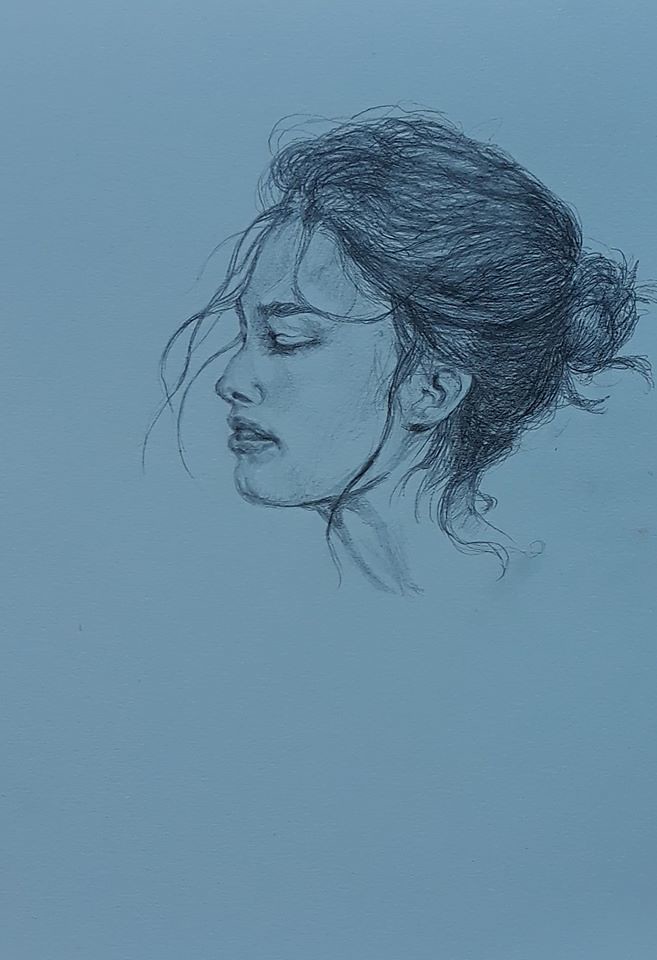This is an intricate ink drawing portraying a profile view of a woman's face and neck. The background is a soft shade of periwinkle blue, adding a serene ambiance to the artwork. The woman features full, expressive lips and a long, elegant neck. Her nose, characterized by a slight bump, is drawn with delicate precision, and her eyes are depicted as gently closed. A striking feature of the portrait is her pronounced eyebrows, which frame her face beautifully. Her dark hair is styled in a tight bun at the back, with numerous loose tendrils cascading around her face, suggesting a breeze's gentle touch. A delicate ear is gracefully visible, adding to her refined appearance. Subtle shadows accentuate the contours of her neck and the underside of her jawbone, enhancing the depth and realism of this striking illustration.